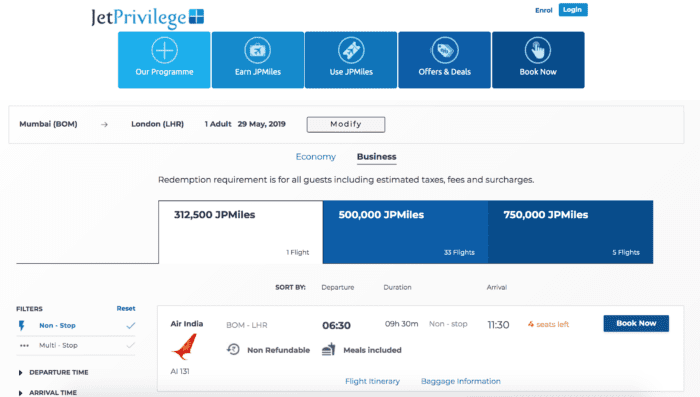The image portrays the homepage of the JetPrivilege website. In the top left corner, the JetPrivilege logo is prominently displayed. The logo comprises the word "Jet" in black with a capital "J," and "Privilege" in blue, structured as one word.

At the top center, the navigation menu begins. The first button, "Our Programs," is highlighted in blue, followed by "Earn JP Miles," "Use JP Miles," "Offering Deals," and "Book Now." Below the menu, specific travel details are listed: "Mumbai" as the departure city, "London" as the destination, and the travel date "29 of May, 2019" for "One Adult." A "Modify" button is also visible for changing the search criteria.

Under these travel details, there are two tabs labeled "Economy" and "Business," with the "Business" tab selected. The screen further shows that the selected Business class flight requires "312,500 JP Miles."